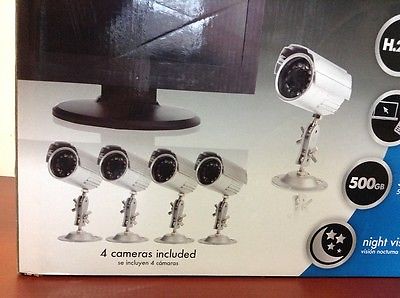This image shows the front of a white and blue box for a security camera system. The box, resting on what appears to be a wooden floor or table with a barely visible white wall behind, prominently features several key elements. On the front, there are images of four small, silver cameras under the text "Four cameras included," reinforcing the contents of the package. The cameras are shown again on the right side of the box. Additionally, the box displays a silver moon with stars icon accompanied by the words "Night Vision," suggesting the cameras' capability to capture footage in low light conditions. A circle indicating "500 GB" is visible, presumably referring to the storage capacity available for the system. Above this, another circle with silver writing is present, and in the top right corner, a circle with a silver letter "H" is seen. In the upper left corner, an image of a laptop is depicted, possibly illustrating the system's monitoring capability. The entire picture has been captured, showing the square-shaped box on a wooden surface.